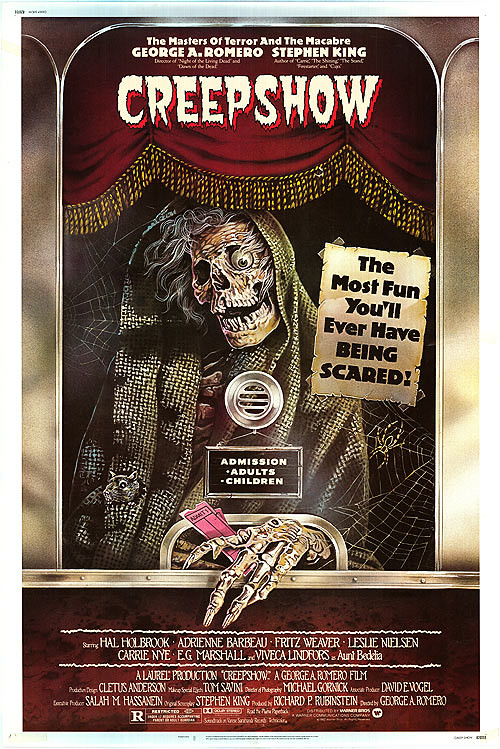A theatrical movie poster for "Creepshow" prominently features a chilling scene within a movie ticket taker booth. Above the booth, a plush red curtain with gold fringes displays the text "The Masters of Terror and the Macabre, George A. Romero, Stephen King" in white font. The title "Creepshow" is also emblazoned on the curtain. Inside the booth, a sinister skeleton wears a tattered cloak with a hood pulled over its head, revealing a grinning visage with one eye and gray hair. The skeleton's bony hand protrudes from the booth, holding two red admission tickets. A spider web with a spider adds to the eerie atmosphere on the right side. A sign taped to the booth's window reads, "The Most Fun You'll Ever Have Being Scared," and the window also displays "Admission, Adults, Children." At the bottom of the poster, the movie credits are listed, including names of actors such as Adrienne Barbeau and Hal Holbrook.